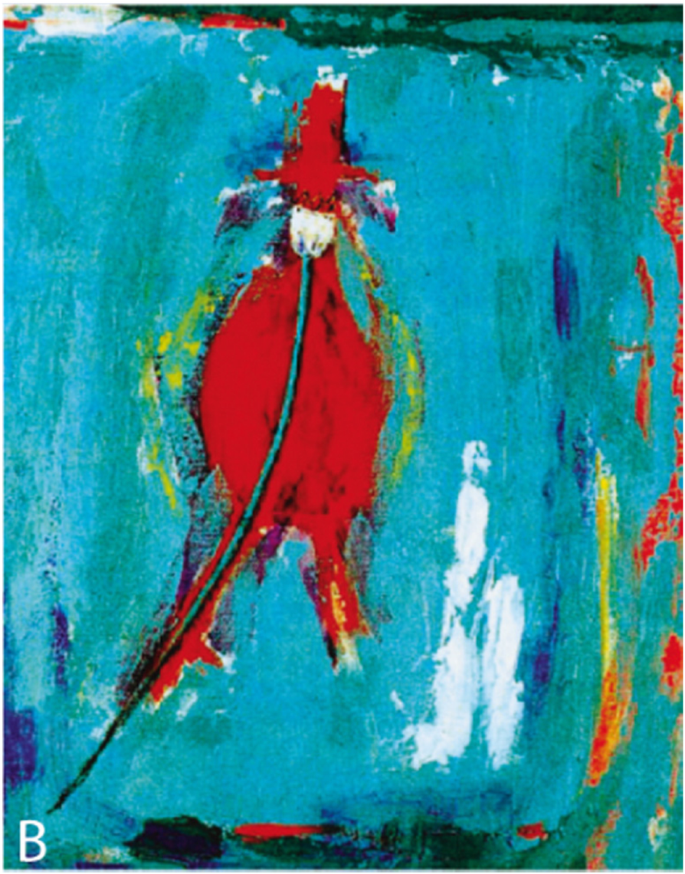This is a highly abstract and pixelated painting characterized by its cyan and teal blue-green background, accentuated with stylized brush strokes and a diverse palette of colors. The central focus of the artwork is a amorphous red shape that can be interpreted in multiple ways: it could represent a fox without arms, a horse-like head with a body resembling a dog, or even a dragon-like creature with a bloated midsection. This red form features legs of different lengths and an elongated stripe extending from its top, which various viewers have likened to a leash or a tongue. Further color details include a dark forest green streak at the top, vibrant crimson streaks, a single yellow streak on the right edge, and darker tones like forest green and navy blue at the bottom. The bottom left corner contains a digitally-added white letter "B" in a typed font. The painting features streaks of white, yellow, and red dispersed throughout, contributing to its dynamic and abstract quality.